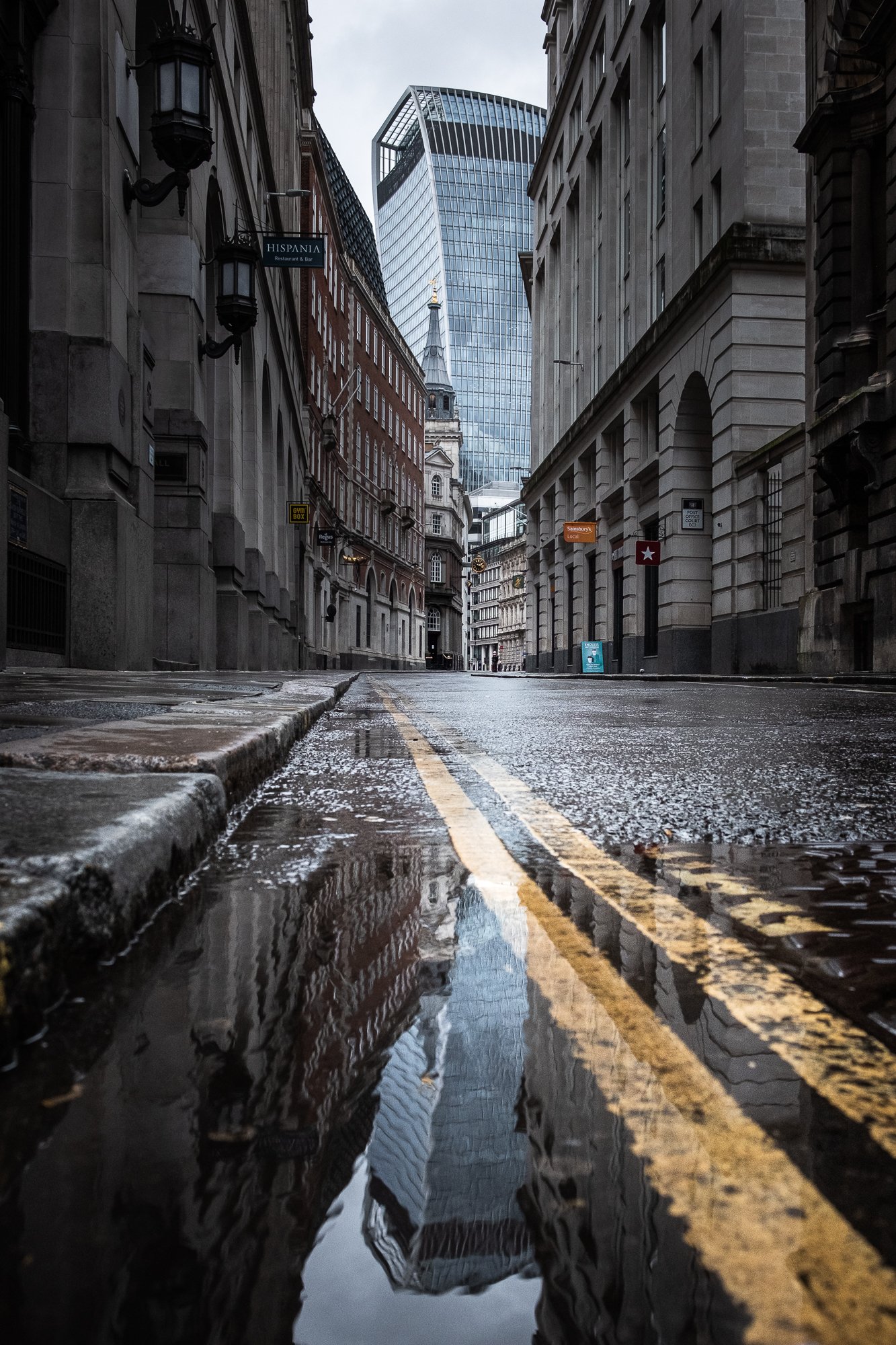The image captures a wet, empty urban street scene taken from a street-level perspective, hovering close to a puddle on the road. Tall gray buildings with slightly old architectural elements line both sides of the road, highlighting a distinctive urban setting. A notable blue sign reading "Hispania" is visible above a pair of lantern top outdoor lights on the right-hand side building. The centerpiece of the background is a large, glass-fronted skyscraper framed by these older buildings. The street itself features an unusually positioned double yellow line, very close to the sidewalk on the left side. The overcast sky reflects in the puddle, adding to the moody and somewhat surreal atmosphere of the scene. There are no people, animals, or creatures in sight, further emphasizing the serene emptiness after what seems to be a recent rain.